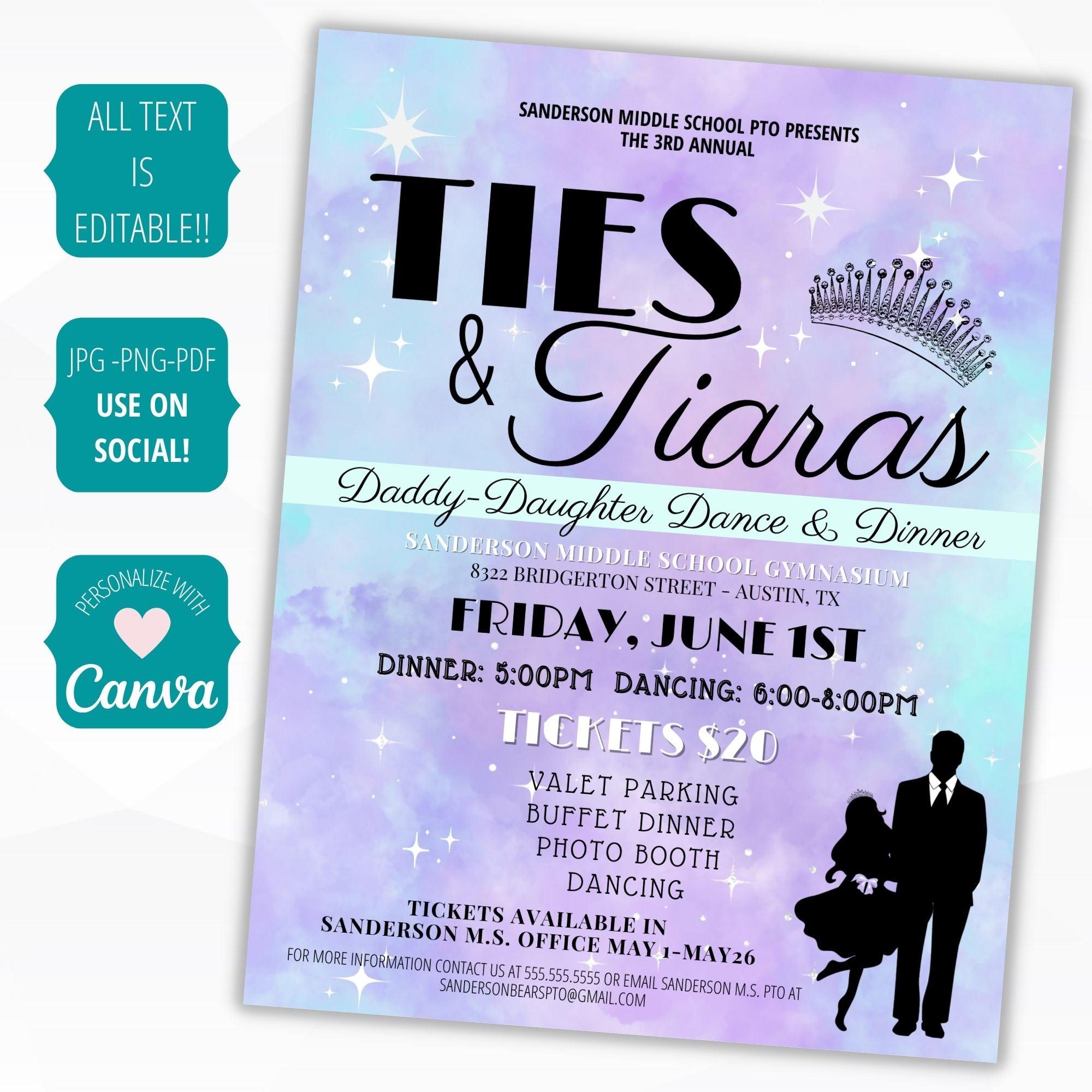The image portrays a white-background digital render of a vividly colored flyer for the "Sanderson Middle School PTO Presents the 3rd Annual Ties and Tiaras Daddy, Daughter, Dance and Dinner." The right side of the flyer, with a blue and purple sky-themed backdrop adorned with white stars of various sizes, displays the main content. At the top, small black fonts read “Sanderson Middle School PTO Presents the 3rd Annual,” followed by the prominent “Ties and Tiaras” title featuring a tiara logo. The tagline, “Daddy, Daughter, Dance and Dinner,” appears beneath.

Further details include the event’s venue at "Sanderson Middle School Gymnasium," located at "8322 Bridgerton Street, Austin, TX," and the event date, "Friday, June 1st." The schedule specifies, "Dinner, 5 p.m.," and "Dancing, 6 to 8 p.m.," with tickets priced at $20. Additional amenities such as "Valet Parking," "Buffet Dinner," "Photo Booth," and "Dancing" are also highlighted. The flyer mentions that tickets are available from May 1 to May 26 at the Sanderson MS Office and provides a contact phone number and email for further information.

Adjacent to the flyer’s main content is a stencil image of an adult male and a young girl. The man, in black shadow, wears a black suit, tie, pants, shoes, and a white shirt. The girl, who is shorter than the man’s shoulder height, sports a black outfit with a skirt, crown, and ribbon at the waist. She strikes a playful, dancing pose with one leg lifted. 

To the left side of the flyer, small green boxes contain editable text options for the flyer, indicating formats available (JPG, PNG, PDF), usage advice for social media, and a note to personalize with Canva, accompanied by a heart symbol.